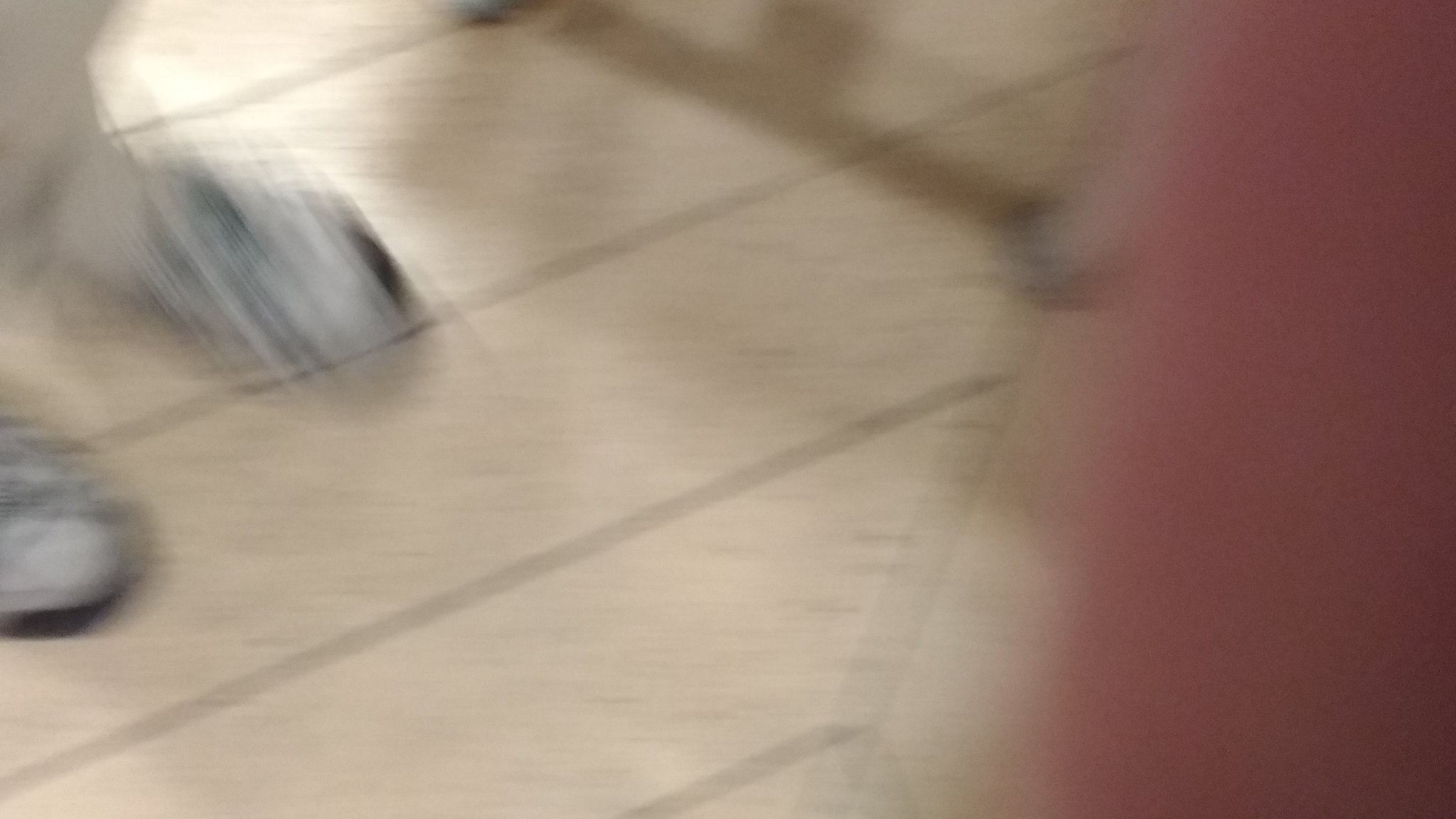The image is highly blurry, making it difficult to discern details clearly. However, it appears to depict a floor made of white tiles with black lines and dotted patterns running diagonally across the image. In the upper left corner, two sneakers are faintly visible; they seem to be gray and dark gray with possible black tips and some brown lines on them. There is also a shadow, likely from a table, casting an additional layer of ambiguity on the top portion of the image.

On the right side of the image, a pinkish object, potentially resembling skin or a hand, partially obscures the view. Nearby, there's a black-handled, pink object which might be merging with the blurry pinkish area. The image is illuminated brightly, suggesting good lighting in the room, and there is a faint outline of white pants and possibly white socks visible among the background items, which blend into the overall haziness of the scene.